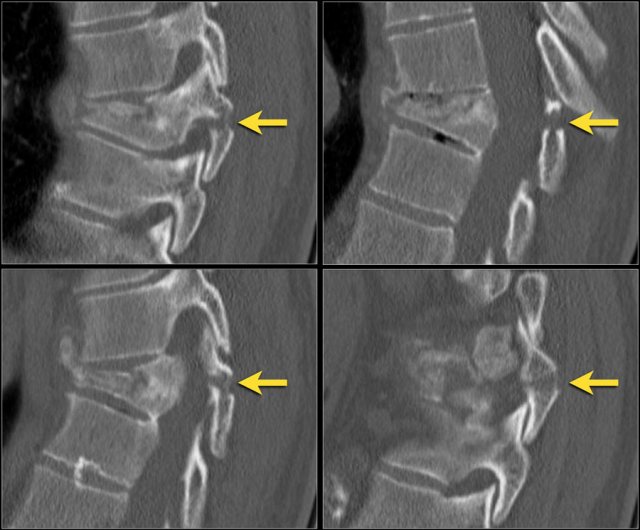The image consists of four separate square x-rays arranged in a 2x2 grid, segmented by a black cross in the middle. The x-rays, predominantly rendered in shades of gray against a black background, depict what appears to be sections of a spinal column. Each x-ray features a yellow arrow pointing to specific parts of the spine, highlighting particular vertebrae or bone structures.

- The top left x-ray shows a segment resembling a spinal column with clear vertebral divisions. The spine extends downward, curving slightly to the left at the bottom, with protrusions on the right side. The yellow arrow here points to a middle section of this spinal representation.
- The top right x-ray also features spinal segments, with a background that transitions from black to gray. The bones appear lighter gray, sectioned, and outlined in white, resembling long ovals. A yellow arrow points to the left between two of these segmented ovals.
- The bottom left x-ray mirrors the upper left image but with larger gaps between the sections. It contains similar protrusions, with the yellow arrow pointing to a specific part that bows out on the right, similar to a kneecap in appearance.
- The bottom right x-ray is less defined and more jumbled compared to the others. It shows a mass of gray with fewer distinct lines, separating near the bottom. Here, a yellow arrow points to a prominent protrusion in the middle right section.

Overall, the image emphasizes detailed sections of the spine, highlighting specific points of interest with yellow arrows in each x-ray.